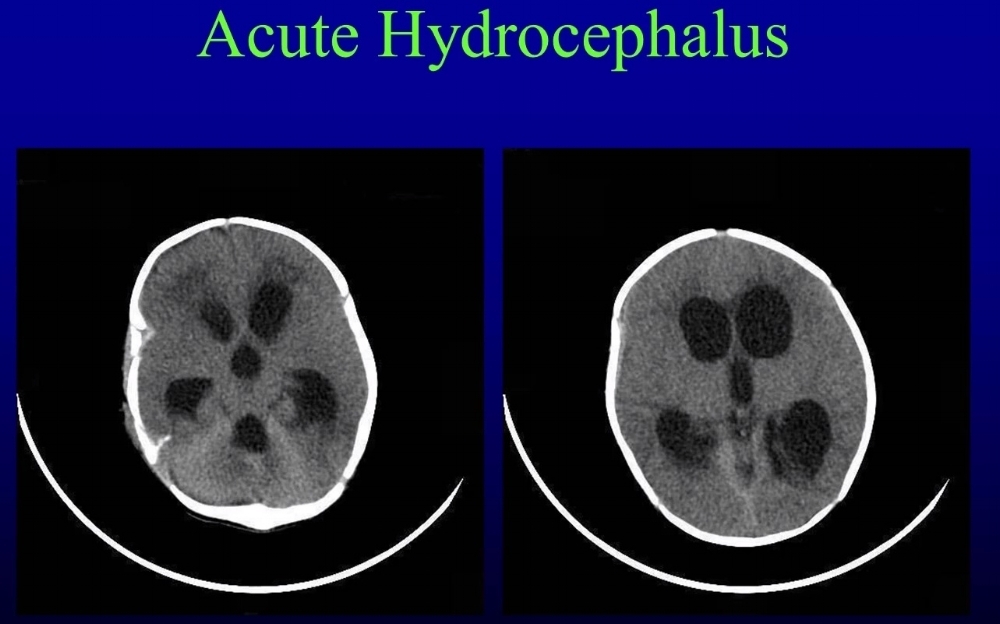The image depicts the medical condition of acute hydrocephalus, prominently labeled at the top in green Times New Roman font against a gradient background that transitions from blue to indigo. Below this title, the image features two x-ray scans set against black squares. These scans display primarily dark gray to light gray brain matter characterized by spongy, vein-like streaks, contained within white-bordered ovals. Additionally, each oval contains five to six small black dots of varying sizes. Beneath each oval is a white semicircle suspending the depicted structures, emphasizing the diagnostic features of acute hydrocephalus captured in these x-ray images.